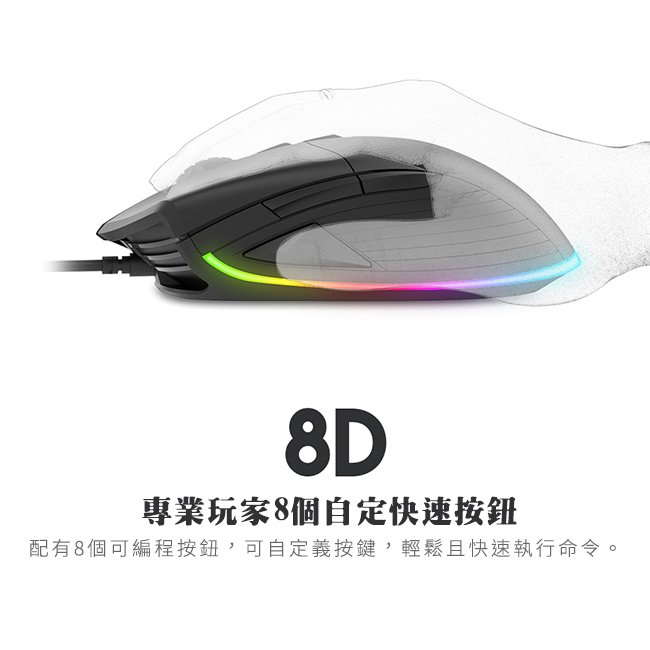This is a detailed, side-view image of a black wired gaming mouse on a white background, likely part of an advertisement. The mouse features a rainbow LED strip along the bottom edge, showcasing vibrant colors that transition through green, yellow, pink, magenta, purple, and blue. Highlighted with various ergonomic details, the design includes multiple side buttons positioned where the thumb would rest, a central scroll wheel, and an ergonomic shape demonstrated by a transparent outline of a hand placed over it. Below the mouse, the large black text reads "8D," followed by smaller black Chinese or Japanese characters, with an additional row of lighter gray characters beneath them. The meticulously crafted design and text positioning enhance its appeal for online retail platforms like Amazon or Newegg.